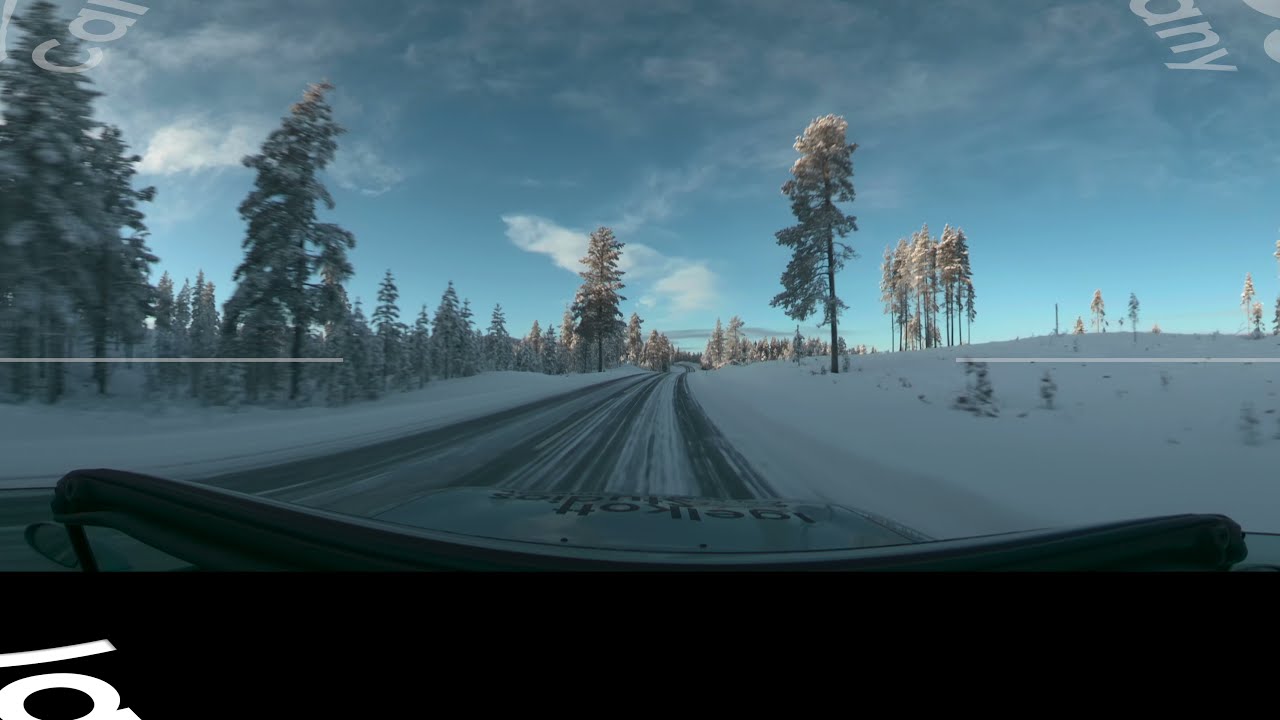The image is a beautiful, wintry scene captured from the dashboard of a vehicle traveling on a snow-covered road. The road, flanked by several inches of snow, stretches into the distance under a sky filled with patches of blue and scattered clouds. On the left side, a dense forest of tall, cone-shaped pine trees reaches high into the air, their branches heavy with snow. The right side features a more sparsely wooded hill, dotted with small plants and a few trees scattered up the incline. Traces of snow remain on the road, marked by faint gray and white lines. The bottom of the image shows the vehicle's hood, covered in gray cloth with dark gray text, and part of the windscreen. Overlaid text is slightly transparent and includes "CAL" in the upper left corner, "ANY" in the upper right corner, and additional shapes and letters along a black bar at the bottom. The scene conveys the serene beauty of a cold winter day, possibly enhanced by a filter that adds a special tone to the photo.